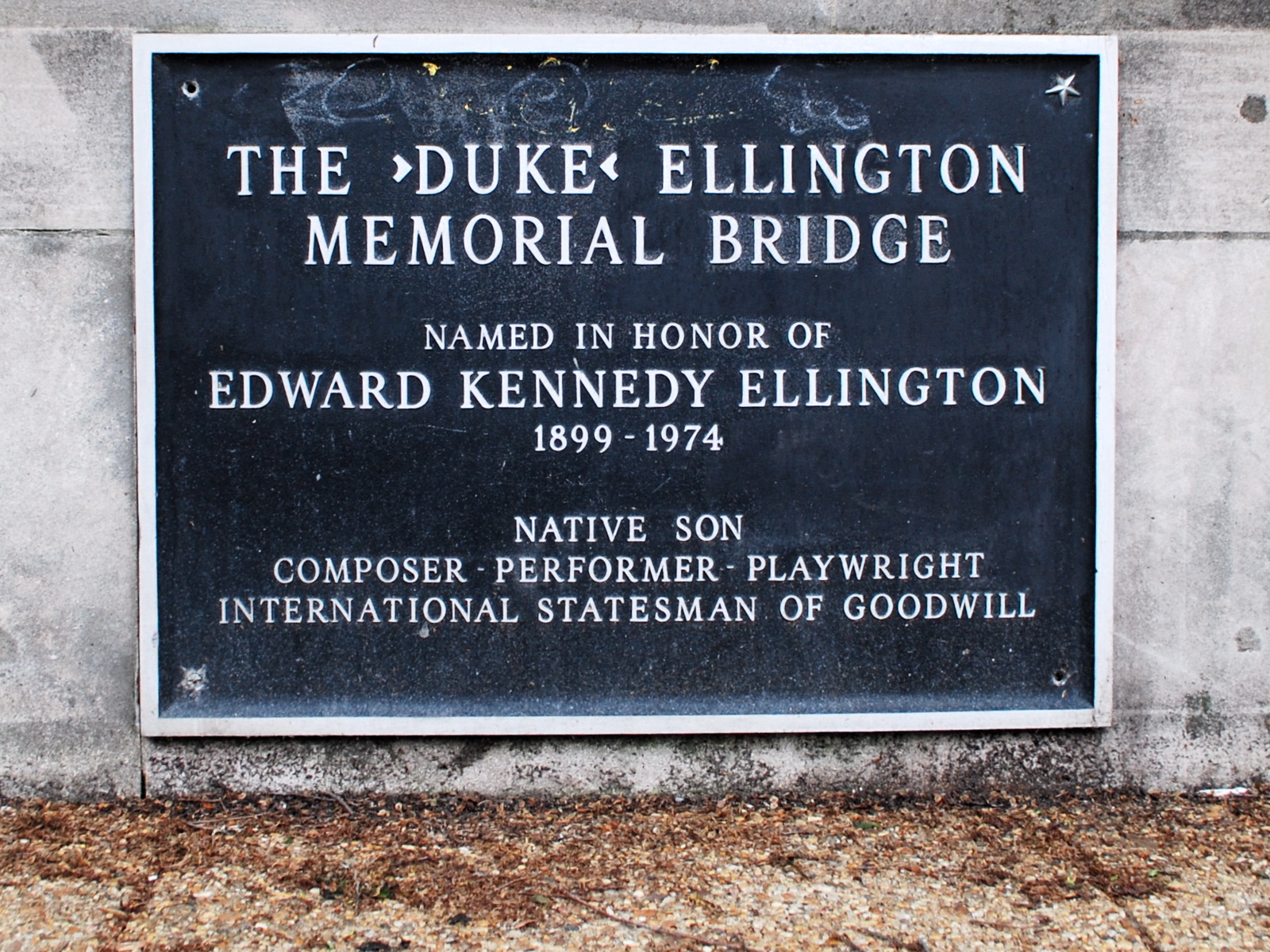This image features a weathered plaque mounted into a concrete wall, likely on the edge of a bridge. The plaque, set within a blue outline and surrounded by a white border, reads in white text: "The Duke Ellington Memorial Bridge, named in honor of Edward Kennedy Ellington, 1899-1974. Native son, composer, performer, playwright, international statesman of goodwill." Notably, a chipped star covers one of the mounting screws in the top right corner, while the remaining corners show empty holes where similar stars once were. The surrounding scene includes a dirt and stone ground, with possibly dirty cobblestone or a gravel walkway near the base of the wall. The setting appears to be outdoors, during the daytime.